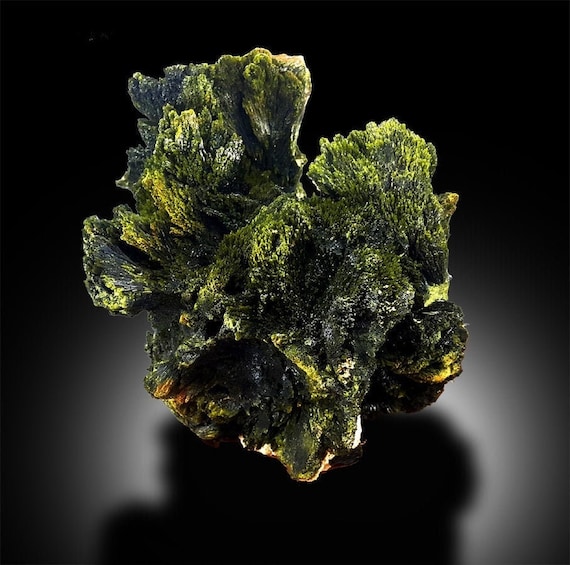This professionally shot close-up photograph captures an irregularly-shaped object, likely a rock, driftwood, or fossil, covered with various shades of green moss. Placed on a smooth, reflective black surface, the object is illuminated brilliantly against an almost entirely black background, which subtly reflects light on its lower half. The rock exhibits a textured, mossy surface with a primary color scheme of deep black interspersed with flecks of green, yellow, and minute patches of white. The moss is more densely concentrated on the upper parts of the object, lending it a vibrant, almost underwater appearance, reminiscent of coral reef structures. The composition highlights the intricate details of the moss and the mysterious, nature-inspired form of the object, creating an intriguing and slightly surreal visual effect.